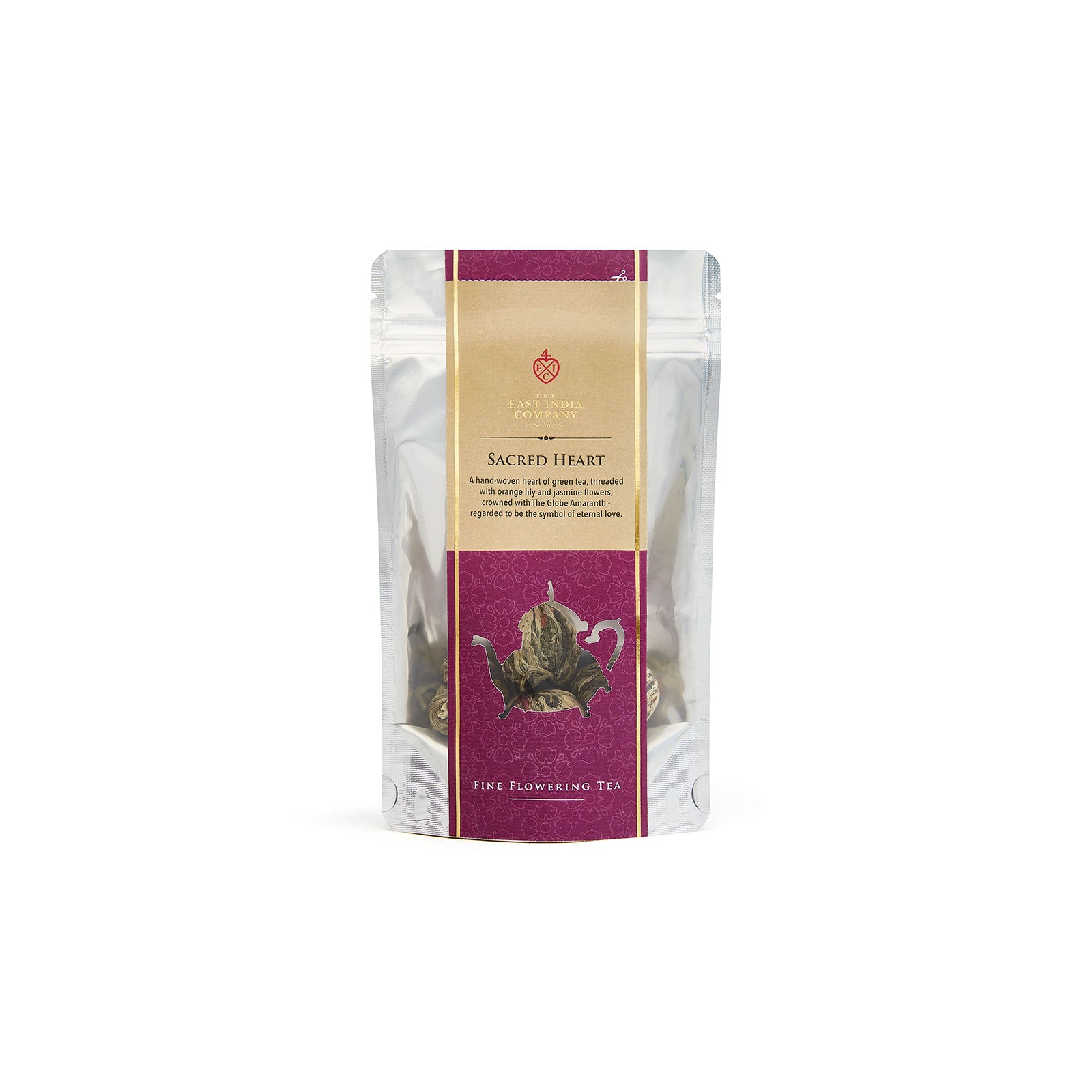This is an image of a sealed, shiny silver tea bag set against a white background. The bag features a prominently placed, long vertical label in a vibrant dark pink (fuchsia) color, adorned with white swirling lines resembling floral shapes. The label is bordered on both sides by thin vertical gold lines. At the top of the label, a light brown, almost caramel-colored box contains a red symbol. Below the symbol, in gold text, it reads "East India Company," followed by "Sacred Heart" in black text. Below this, in black italicized font, there is some writing that is difficult to discern from the provided distance. Further down, the label displays an image of a teapot. Beneath the teapot image, in white text, the label reads "Fine Flowering Tea." The bag is a foil pack with a transparent side, allowing the tea leaves within to be partially visible, including clumps of the fine flowering tea.